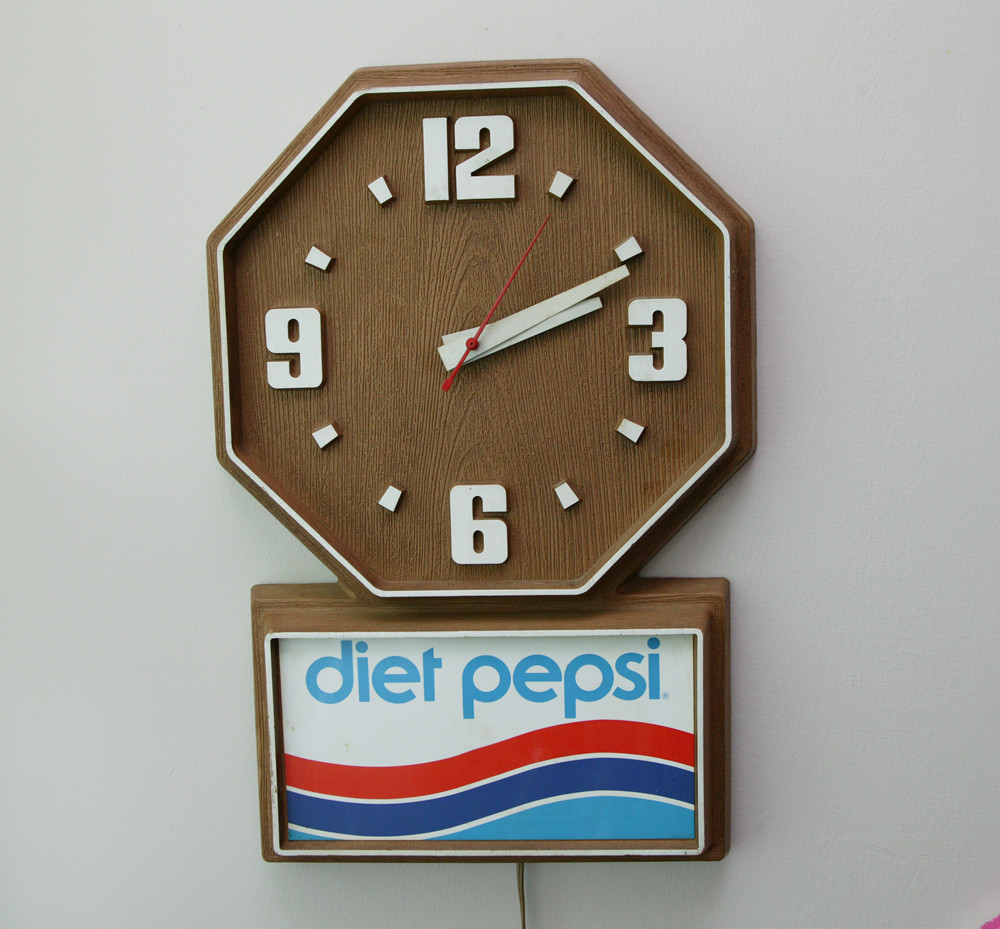The photograph depicts a clock hanging on a white wall. The clock, shaped like a stop sign, is an octagon with a light brown, wood-like material and white trim. It features big, bold, white numbers at the 12, 3, 6, and 9 positions, while the remaining hours are marked by small white dashes or squares. The clock's hands are white, with the seconds hand being a thin red line, indicating the time as approximately 2:11 or 2:12. Attached below the octagonal clock is a rectangular framed Diet Pepsi advertisement, crafted from the same brown material as the clock. The sign includes the Diet Pepsi logo in blue script on a white background, with waves of red, dark blue, and light blue below it. A wire extends down from the clock to the frame of the sign.